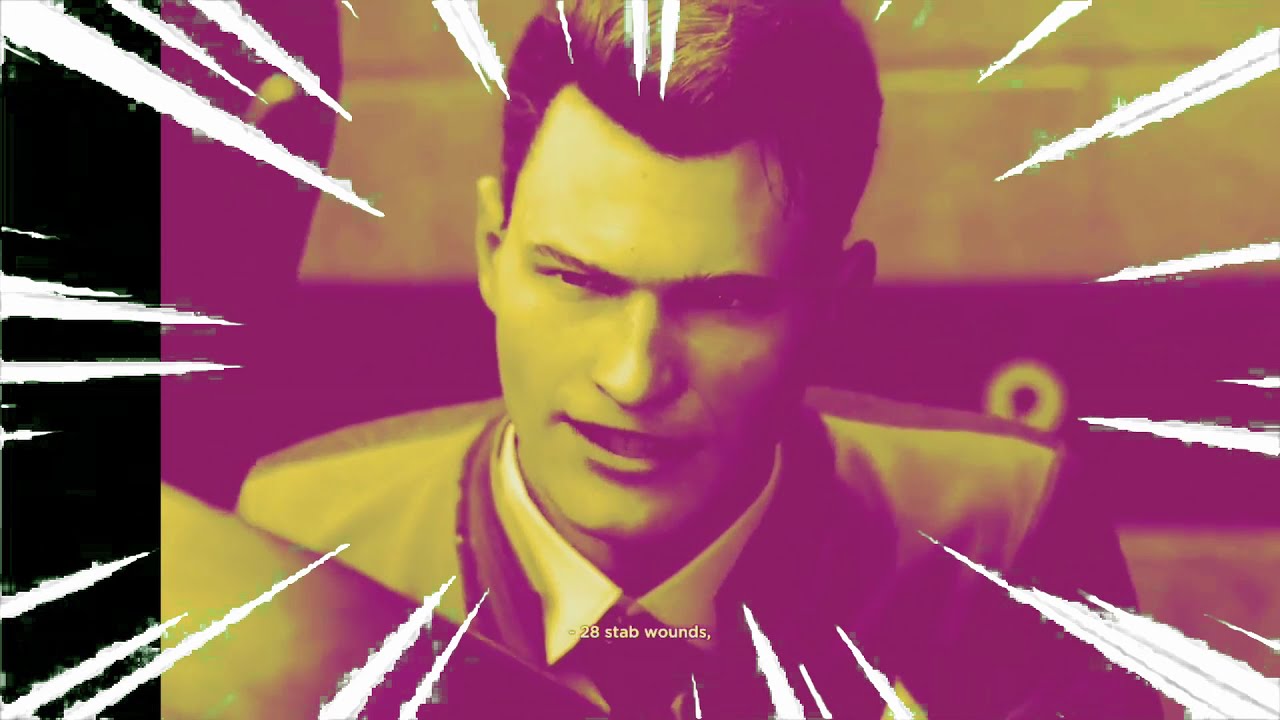The digital artwork appears to be a widescreen, rectangular image heavily shaded in yellow and purple hues. Dominating the center is a 3D-rendered man shown from the shoulders up, wearing a suit and a collared shirt. His face, featuring brown hair that's slightly balding, displays a confused expression with his mouth open, as if he's exclaiming something. The backdrop consists of a wall segmented into large tiles. His visible ears are framed by sharp, white, jagged triangular lines that point inward, conveying intense emotion or shock. On the left side, there is a noticeable black strip. In the background, we can see the back of another character’s head, suggesting a conversation. At the bottom of the image, a subtitle reads "28 stab wounds" in small white font, indicating an impassioned dialogue scene. The dramatic color scheme and the dynamic linework emphasize the tension and gravity of the moment, reminiscent of a stylized video game cutscene.